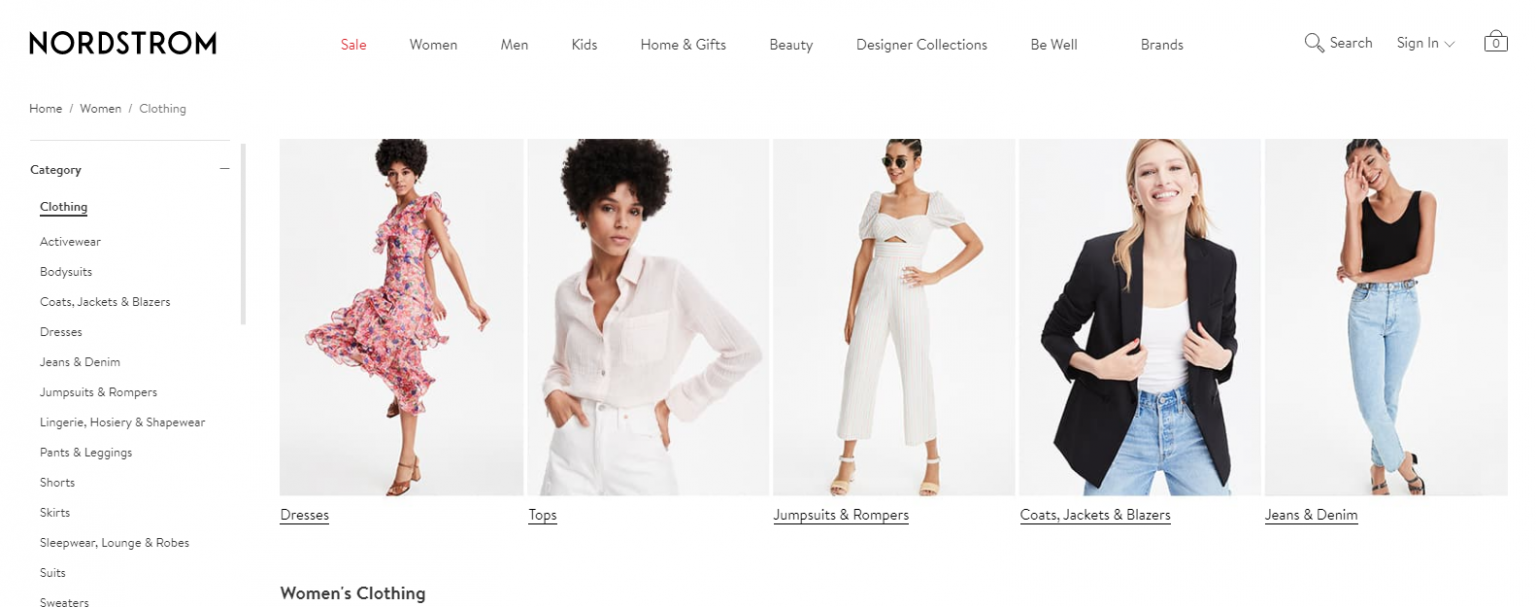This screenshot from a Nordstrom shopping site presents a well-organized interface for navigating various product categories. In the upper left corner, the Nordstrom logo is prominently displayed. Across the top right of the page, several categories are listed in a horizontal menu: "Sale" (highlighted in red), with "Women," "Men," "Kids," "Home & Gifts," "Beauty," "Designer Collections," "Be Well," and "Brands" displayed in black text.

Beneath this menu is a search bar, flanked by a "Sign In" option and a shopping bag icon. On the left side of the page, a vertical navigation menu allows users to drill down into specific categories starting from "Home" and "Women" to "Clothing," which is further subdivided and highlighted. Under "Clothing" are various subcategories, including Activewear, Bodysuits, Coats, Jackets & Blazers, Dresses, Jeans & Denim, Jumpsuits & Rompers, Lingerie, Hosiery & Shapewear, Pants & Leggings, Shorts, Skirts, Shapewear & Lounge, Suits, and Sweaters.

To the right, the main section displays five images corresponding to different clothing categories. The first image depicts an African American woman with black hair wearing a pink dress. The next image shows the same woman in an off-white shirt paired with white pants, labeled "Tops." The subsequent image labeled "Jumpsuits & Rompers" features the woman in a white romper. The fourth image, labeled "Coats, Jackets & Blazers," showcases a Caucasian woman with blonde hair in a black jacket. Finally, the "Denim & Jeans" section shows a woman in a black tank top and light blue jeans.